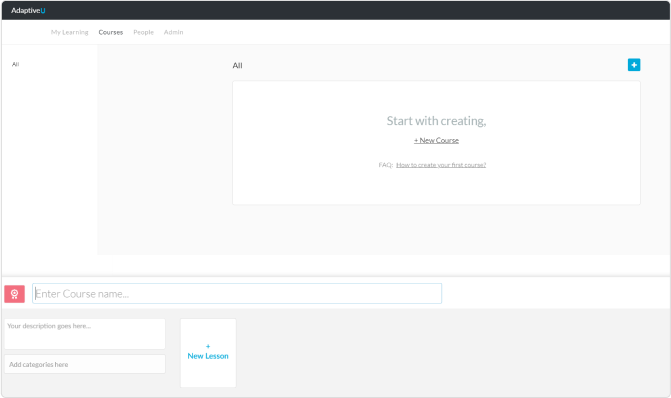A screenshot from the Adaptive U platform is depicted. At the top of a black banner, the platform's name "Adaptive U" is prominently displayed, with "Adaptive" in white font and "U" in blue. The interface's navigation menu is visible, featuring tabs titled "My Learning," "Courses," "People," and "Admin." The "Courses" tab is selected and highlighted in bold. 

Beneath the banner, there's a section labeled "All" written in black text on a white background. Adjacent to it is a square blue button with a plus sign. In the center of the screen, a blue square button reads "Start with Creating." Another highlighted section reads "New Course," accompanied by a plus button.

Various interactive elements populate the interface, including a "Facts, FAQ" section that guides users with a hyperlink titled "How to Create Your First Course," which is underlined for emphasis. Additionally, a red rectangular button labeled "Enter Course Name" is present, indicating where the course title should be input. A box titled "Your Description goes here" prompts users to add a course description. Another box invites users to "Add Category here." Lastly, a blue square box titled "New Lesson" indicates the starting point for adding lesson content.